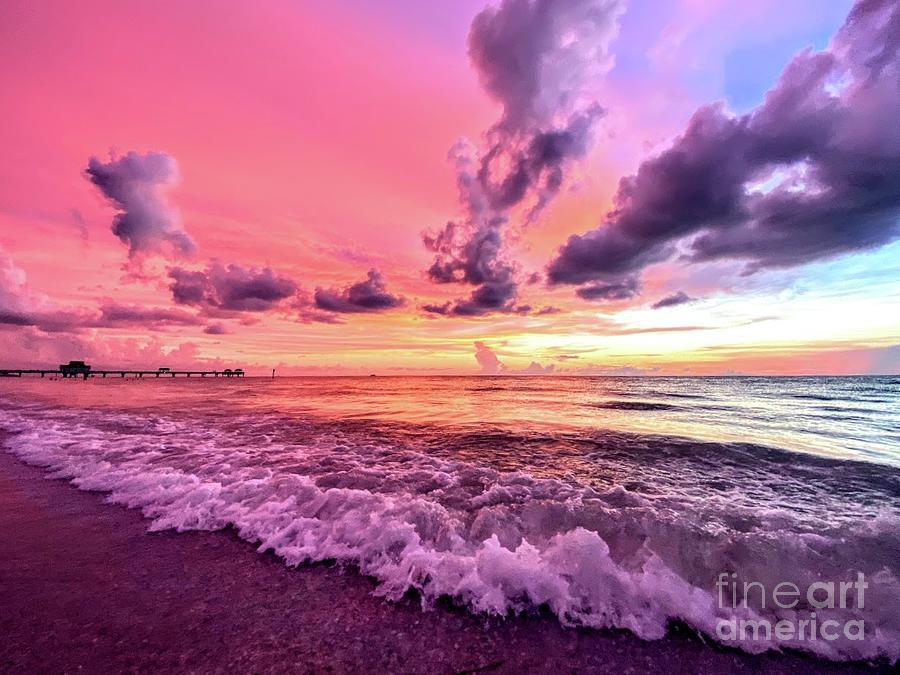This is a stunning, highly detailed photograph of a beach at sunset, captured from a very low angle to emphasize the natural beauty and ambiance of the scene. On the bottom left corner, the sandy shoreline features small waves lapping against it, with some white foam visible. A dark silhouette of a pier or boardwalk juts out into the water, accompanied by a distant boat and a large structure on the pier in the center of the image. The sky is a vibrant mix of colors, with the upper left side displaying hues of pink, orange, and purple, while the upper right side transitions into blue tones. Gray and dark clouds are interspersed across the sky, which, in combination with the low sun and light diffraction, creates a mesmerizing sunset. The water reflects the sky's colorful gradient, adding to the serene atmosphere. A watermark in the bottom right corner reads "Fine Art America," identifying the source of this beautiful and realistic piece of art.